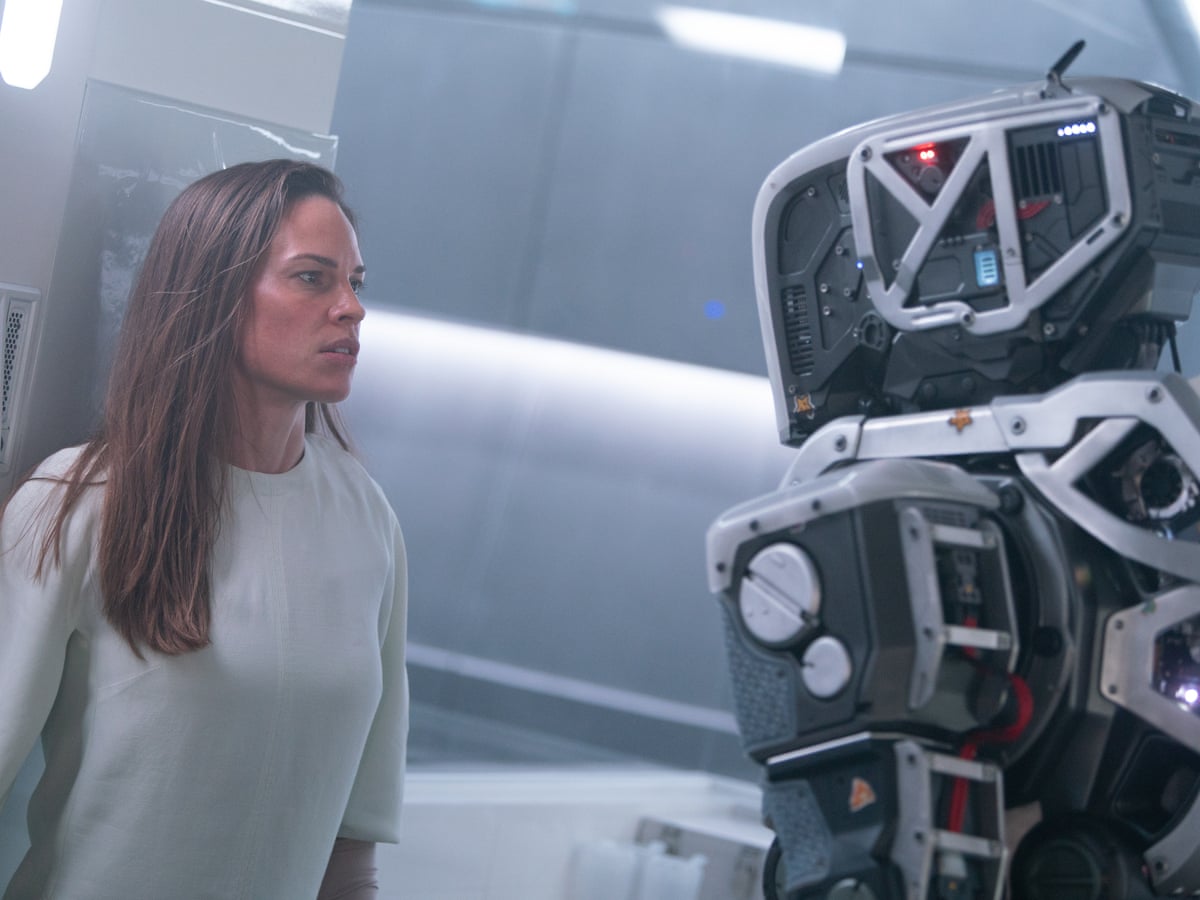In a stark, futuristic room with bright white tiles and white lighting, A-list actress Hilary Swank leans against a white column, her face a mix of fear and worry. Dressed in a plain, long-sleeved white blouse, her brown hair falls straight and past her shoulders. She stares intensely to her right at a menacing, humanoid robot. The robot, which appears designed for intimidation, is composed of black components bordered in silver and white. Its rectangular head and body are adorned with numerous LED lights and electrical cords, highlighting its advanced, high-tech nature. The tension in the scene suggests an impending standoff between Swank and the machine, portraying a dramatic moment likely captured from a movie.